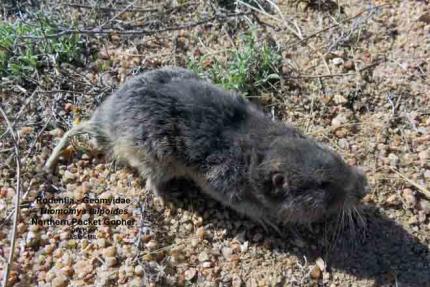This close-up photograph captures a small rodent, identified as a northern pocket gopher, in its natural outdoor habitat. The gopher has a gray coat of fur with a white underbelly and is characterized by its slender, long tail, small ears, and prominent whiskers. It also features long claws on its front feet. The image is set during the daytime, as indicated by the shadow cast to the right by the gopher's head. The ground is composed of gravel and sand, interspersed with patches of green vegetation and scattered twigs. The rodent is caught in motion, moving from the left to the right side of the photo, with its surroundings suggesting a desert-like environment. In the bottom left corner, there is partially visible text that includes the word "rodentia." The central focus of the image is clearly the gopher, highlighting its detailed features and natural setting.